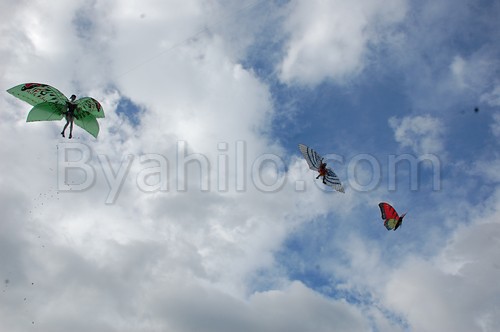In this whimsical scene, a blue sky is interspersed with fluffy white clouds, creating a dreamy backdrop. Overlaid in semi-transparent white font is the text "byahilo.com". The focal point of the image features three fantastical butterfly-like figures. The most prominent has a human-like body with large, green wings adorned with subtle black etchings, positioned above the letter 'B'. Another figure with similar fairy-like characteristics and black-striped wings is found over the 'C'. A third butterfly with red and yellow wings is situated below the letters 'O' and 'M'. The butterflies, varying in their movements, appear not to interact with each other, adding to the magical, serene quality of the scene.